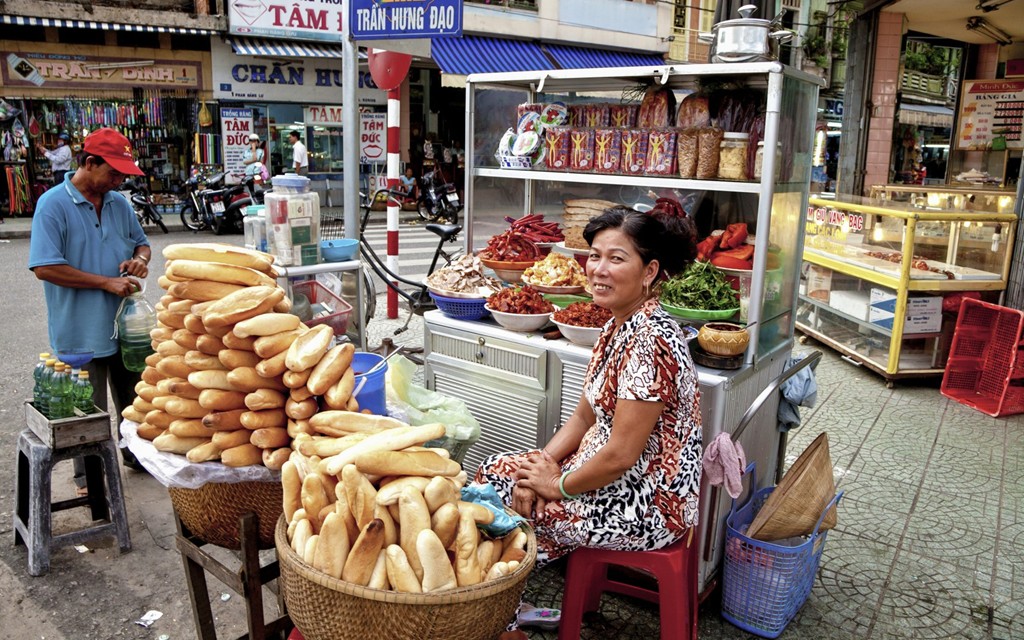This photograph captures an outdoor street market scene, likely in Vietnam, as indicated by the "TRAN HUNG DAO" street sign in the background. At the center of the image is a woman with dark brown hair, smiling at the camera and wearing an animal print dress while sitting on a red stool. In front of her, two wicker baskets are filled with elongated baguette-like loaves of bread. Behind her is a metal cart adorned with an array of colorful bowls containing various foods, including meats and greens in different styles, and several types of vegetables, possibly peppers. Additional containers above these bowls hold an assortment of snacks, which might include nuts. To the left, a man in a blue collared shirt and a red baseball cap holds a water bottle, with more bottled water on a nearby bench. In the background, gold and glass cabinet casings are visible in front of a storefront, and across the street, several shops are lined up, including one with a blue sign that reads "CHAN HUG" and another with a red sign that says "TAM." This bustling market scene provides a vivid glimpse into the local street culture and commerce.